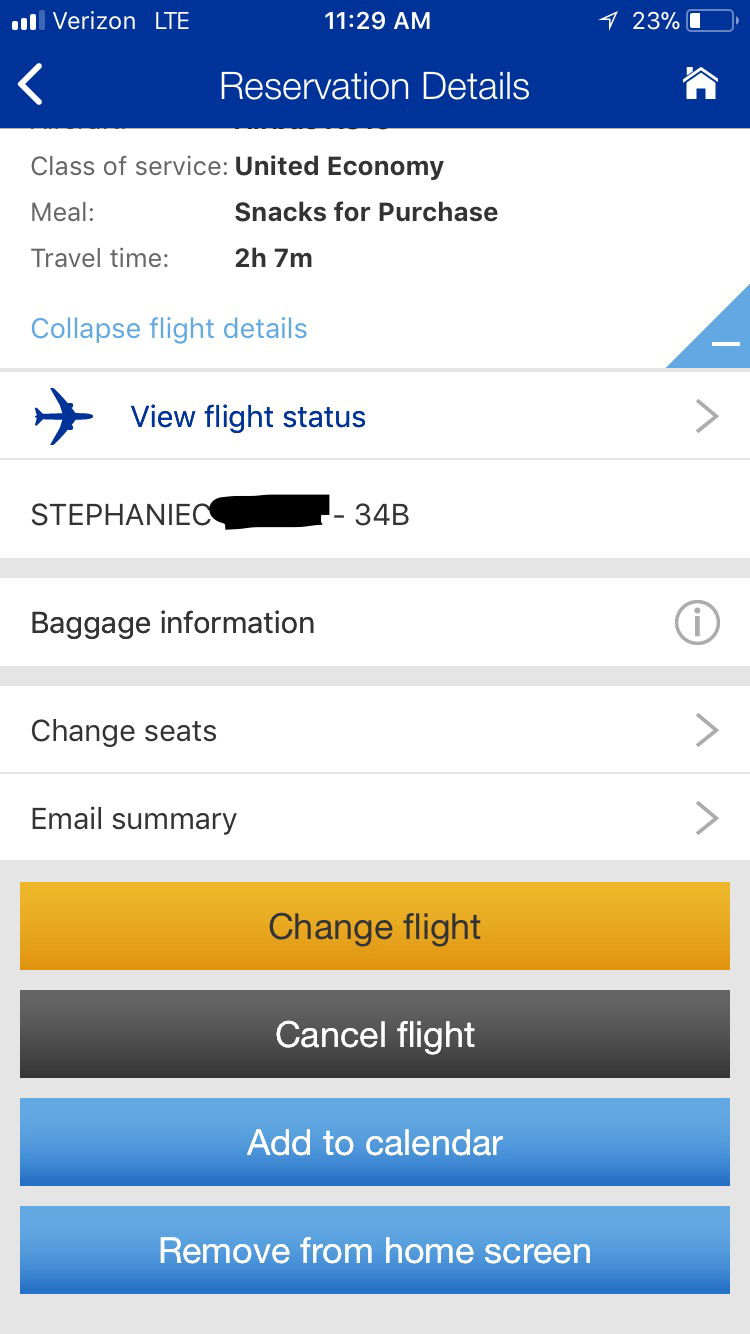The image features a mobile application interface set against a white background. At the top, there's a prominent blue header displaying essential information such as "Verizon LTE," the current time "11:29 AM," and battery status "23%". Additionally, icons for a left arrow, "Reservation Details," and a home symbol are present.

Below the header, the white background continues with detailed flight information. It indicates the "Class of Service" as "United Economy," notes that "Meals" and "Snacks for purchase" are available, and lists the "Travel time" as "2 hours and 7 minutes." There is also an option to "Collapse flight details" at the bottom of this section. In the bottom right corner of this segment, there is a small blue triangle with a white line.

Following this, a series of white boxes with blue accents provide additional functionalities. The first box features a blue airplane icon and the text "View Flight Status" accompanied by a right-facing arrow. The next box displays the passenger’s name, "Stephanie C," with the rest blacked out, followed by the seat number "34B" and a horizontal blue line.

Further down, another white box labeled "Baggage Information" includes an icon of a circle with an 'i' for information. Below it, more white boxes offer options: "Change Seats" with a right-facing arrow, "Email Summary" with a right-facing arrow, and finally, a larger blue section at the bottom.

The concluding blue box contains several functional buttons: a yellow button labeled "Change Flight," a gray button labeled "Cancel Flight," a blue button labeled "Add to Calendar," and another blue button labeled "Remove from Home Screen."